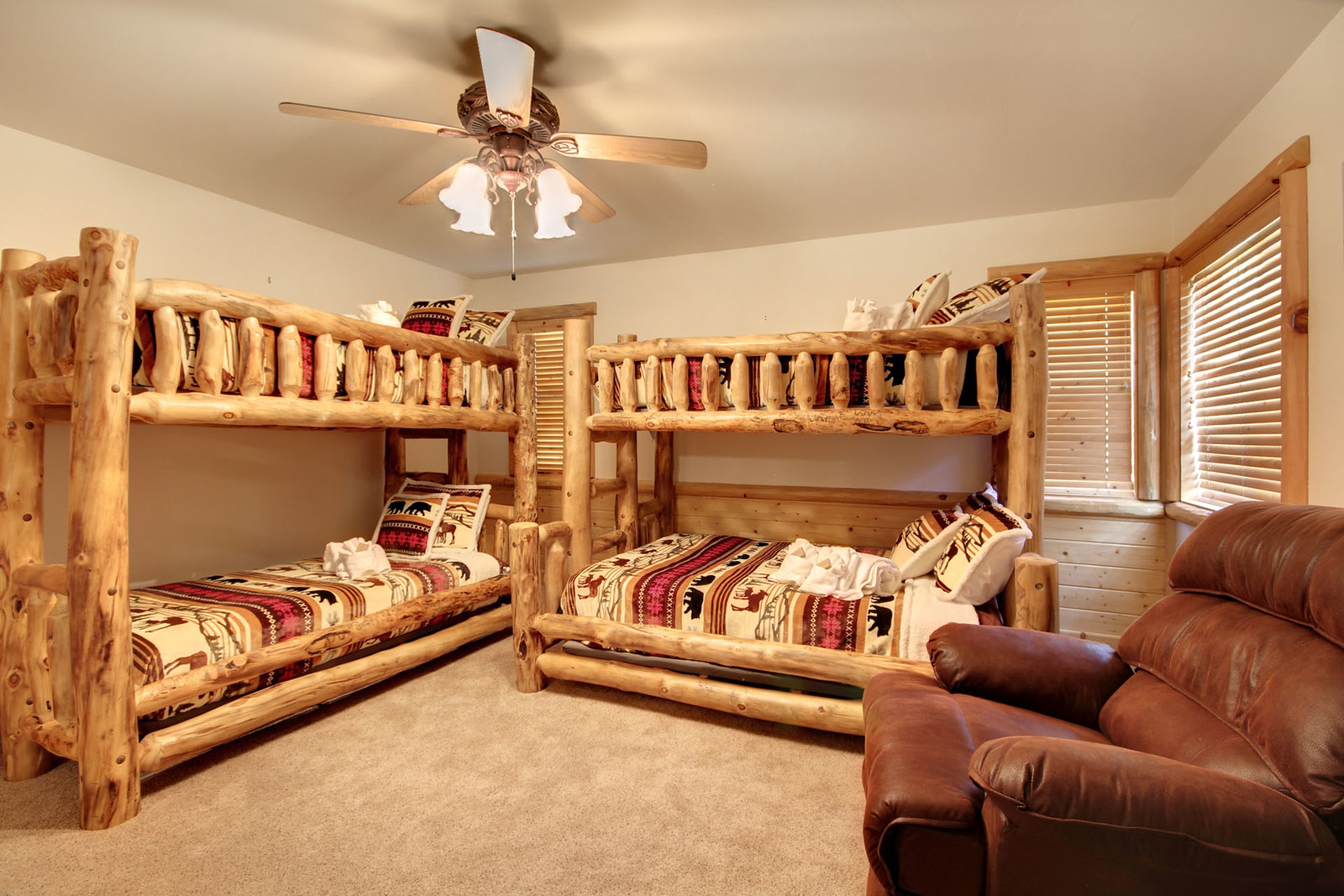This image captures a tidy, well-lit bedroom with a rustic, cabin-like aesthetic. The room features two sets of bunk beds, each constructed from thick, rugged logs that give off a handcrafted feel. These bunk beds have matching, rustic-themed bedding adorned with intricate patterns, possibly inspired by Native American designs, featuring elements like animal motifs and crosses, predominantly in shades of white, yellow, and brown. Each bed is neatly made with two pillows showcasing enhanced sections of the same aesthetic pattern. Towels, likely provided for guests, are folded on the beds.

Suspended from the ceiling is a fan lamp with four illuminated bulbs and pull strings, adding to the room's cozy atmosphere. In the bottom right corner of the room sits a brown leather recliner, enhancing the comfort and inviting feel of the space. The room boasts tan carpeting and white walls, which contribute to its clean and uncluttered appearance. There are two windows in the corner, framed with white wood, allowing natural light to stream in through the basic wooden blinds, harmonizing with the room's overall design and color scheme.